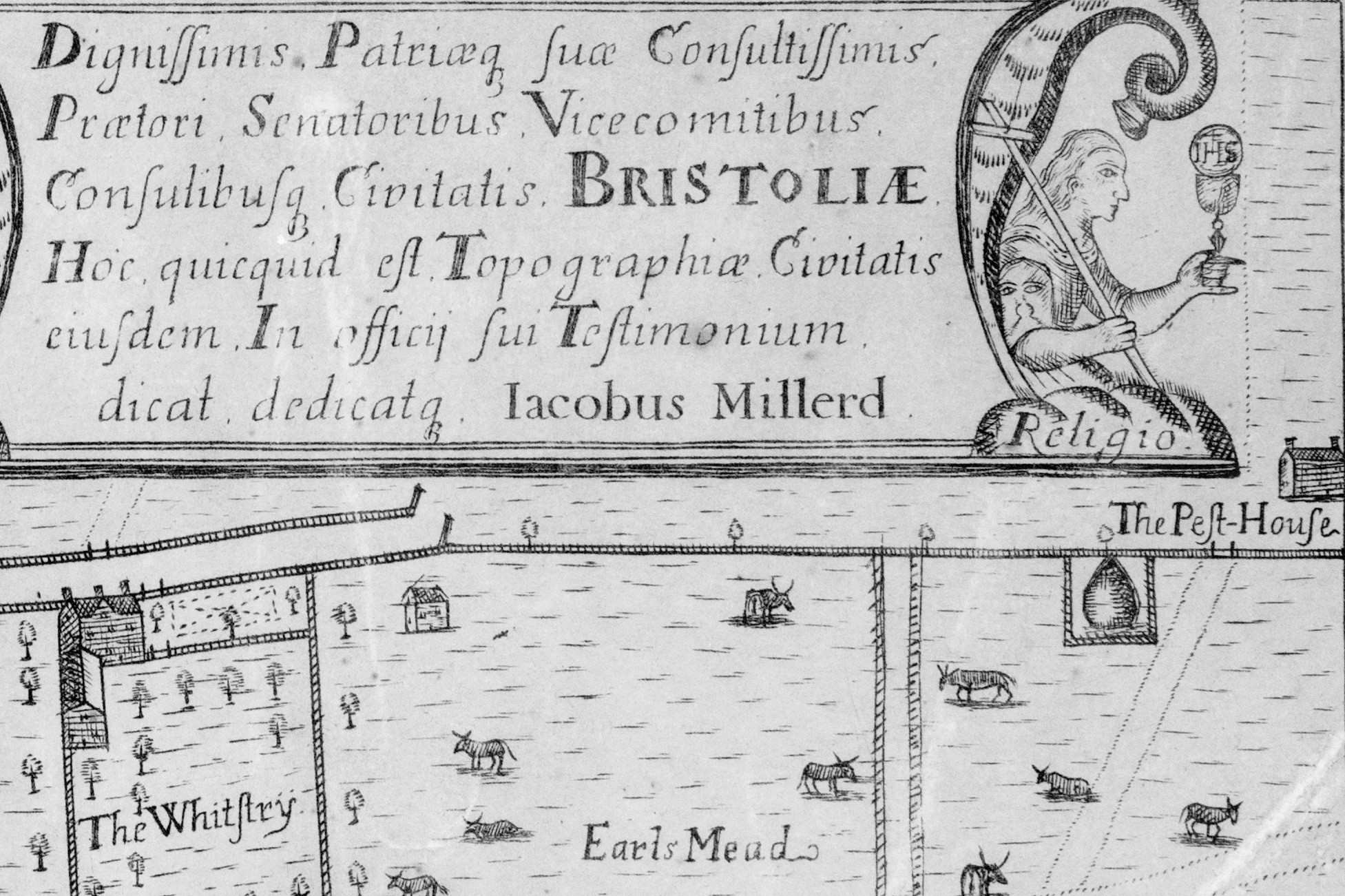The image appears to be a detailed black and white drawing of a medieval-style illuminated manuscript. The top section features extensive Latin text, including a quote attributed to Jacobus Millard. Central to the composition is an illustration of a figure, possibly a religious cleric or priest, seated on a throne of clouds. This person holds a staff with a cross in one hand and balances a goblet on a ball inscribed with the word "religio" in the other. The Latin text surrounding this figure references the words "dignificence" and "Bristoliae." Below this, the manuscript transitions into a meticulously hand-drawn map depicting various farmlands. The map includes labeled areas such as "Whitfrey" on the left and "Earl's Mead" in the center. The right side features a building labeled "Pest House." Scattered across the map are illustrations of cattle and trees, adding to the intricate depiction of the landscape.